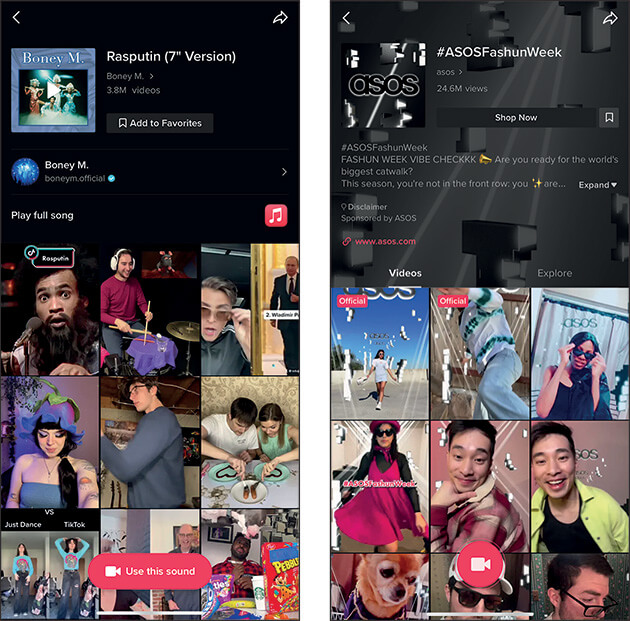This image is a juxtaposition of two different TikTok pages captured side by side. On the left, the TikTok page features content related to the band Rasputin, showcasing various clips that revolve around a song by the band. Below these clips, different TikTok users are seen engaging creatively with the music, performing various activities in time with the song. 

On the right, the TikTok page showcases ASOS Fashion Week, a digital event organized by the popular online retail brand ASOS. The screen captures show numerous individuals participating in fashion try-on hauls, strutting the catwalk, and demonstrating styling tips. The text overlay at the bottom reads, "ASOS Fashion Week - Fashion Week vibe check. Are you ready for the world's biggest catwalk? This season you're not in the front row," positioning viewers to experience the excitement of fashion week from a unique and engaging perspective. Both TikTok pages highlight the dynamic and creative nature of user-generated content on the platform, with one side emphasizing music interaction and the other spotlighting fashion trends.